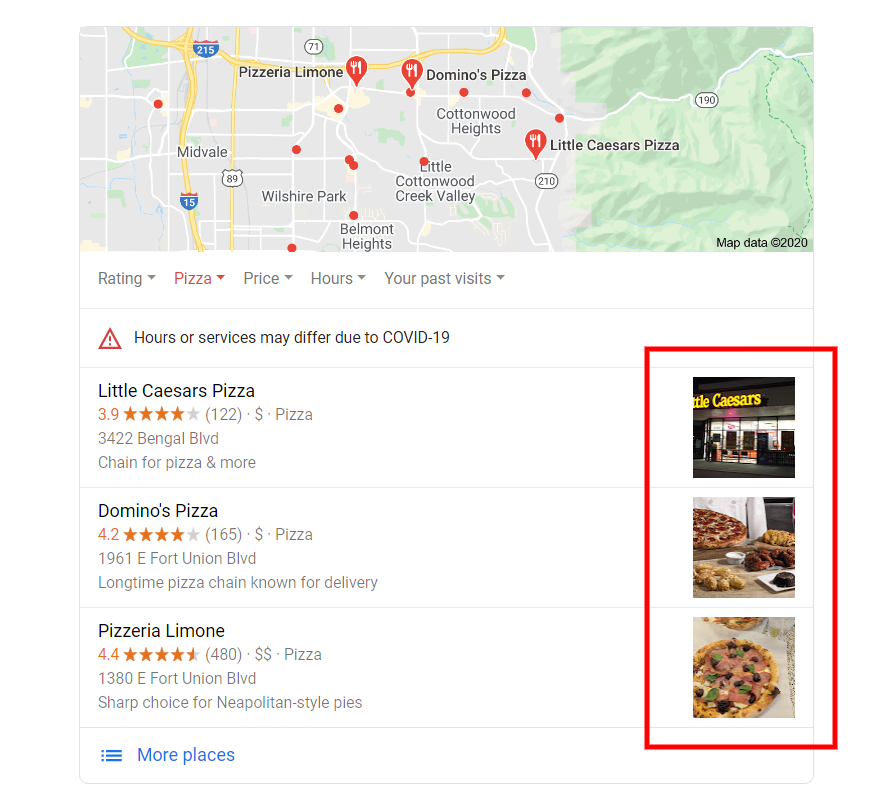This image depicts a detailed map highlighting various pizza places, displayed prominently at the top. The map features three distinct pizza locations, each marked with a red pin icon containing a fork and knife. Below the map, a selection panel offers ratings, pizza options, prices, operating hours, and records of past visits, with "pizza" highlighted in red for emphasis.

Underneath the selection panel is a cautionary message with a triangle and exclamation mark, stating, "Hours or services may differ due to COVID-19." This warning is framed in a red box, indicating the potential for changes.

The listed pizza establishments include:
1. **Little Caesars Pizza** - The entry includes the name, address, a description noting it as a chain for pizza and more, and a photograph of the store's exterior.
2. **Domino's** - Named and addressed similarly, this long-established pizza chain is accompanied by a photo showcasing a freshly made Domino's pizza.
3. **Pizzeria Limone** - Identified with an address and described as a sharp choice for Neapolitan-style pies, along with an appetizing image of one of their signature pizzas.

Overall, this image provides a comprehensive overview of selected pizza places, emphasizing their unique attributes and alerting viewers to possible operational changes due to COVID-19.